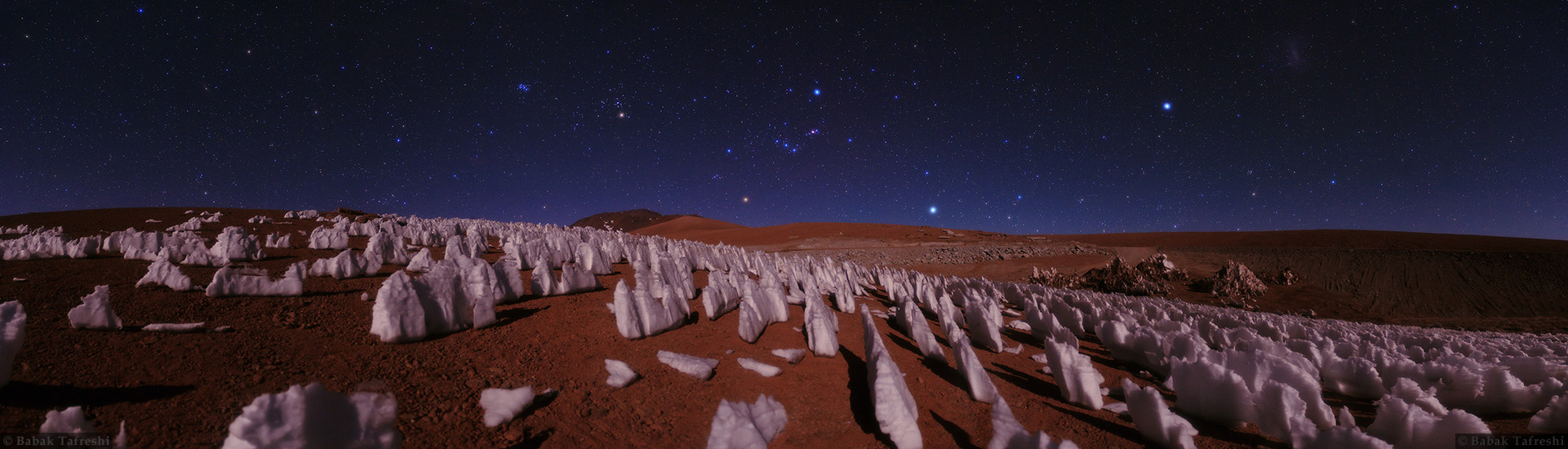A mesmerizing digital rendition showcases a surreal desert landscape under a vibrant, star-studded night sky. The luminous sky features a gradient of dark blue to black, dotted with stars of various hues, including blues, whites, yellows, and subtle purples, suggesting possible color enhancement. Below, the expansive plain of rich, brown soil is punctuated by an array of thin, upright rock formations, resembling crags or monolithic stones. These standing stones, akin to a fantastical depiction, appear to be methodically aligned, yet each maintains a distinct separateness. The stones, which could also be partially buried, extend towards a distant hill that echoes the same unusual formations. This composition creates an otherworldly atmosphere that blurs the lines between reality and imagination, evoking thoughts of an extraterrestrial landscape possibly inspired by the surface of the moon or a far-off planet.